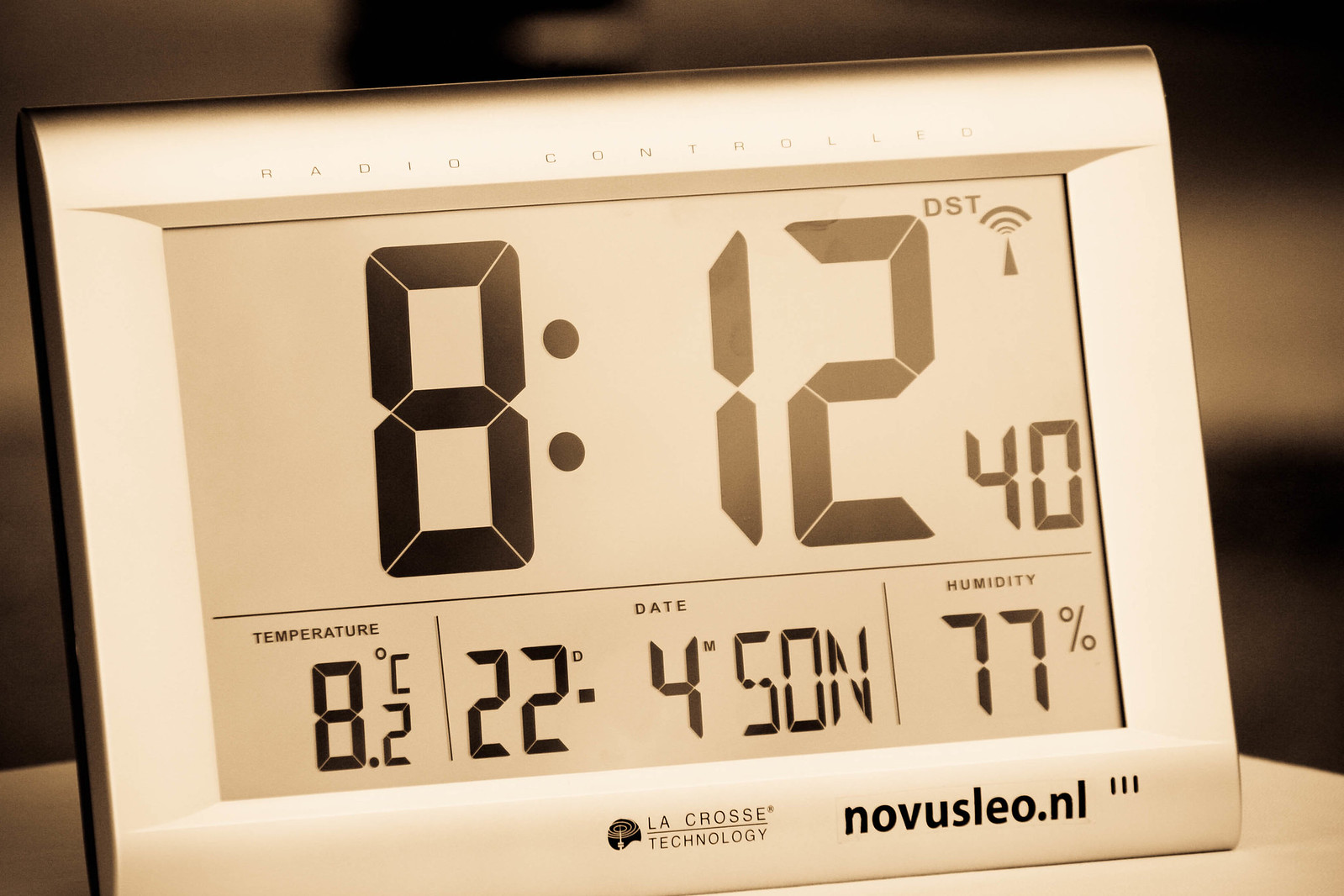The black and white, close-up image captures a digital thermostat from La Crosse Technology. At the top of the device, the small text reads "radio controlled." The bottom of the thermostat prominently displays the La Crosse Technology logo in black ink, with "novuslio.nl" written beside it. The screen exhibits several key readings: a large, bold display of the time as 8:12, a temperature reading of 8.2 degrees Celsius, and the current date format with "22" for the day and "4" with a small "m" indicating April, ultimately reading April 22. Additionally, the thermostat shows a humidity level of 77%, marked underneath its respective button.